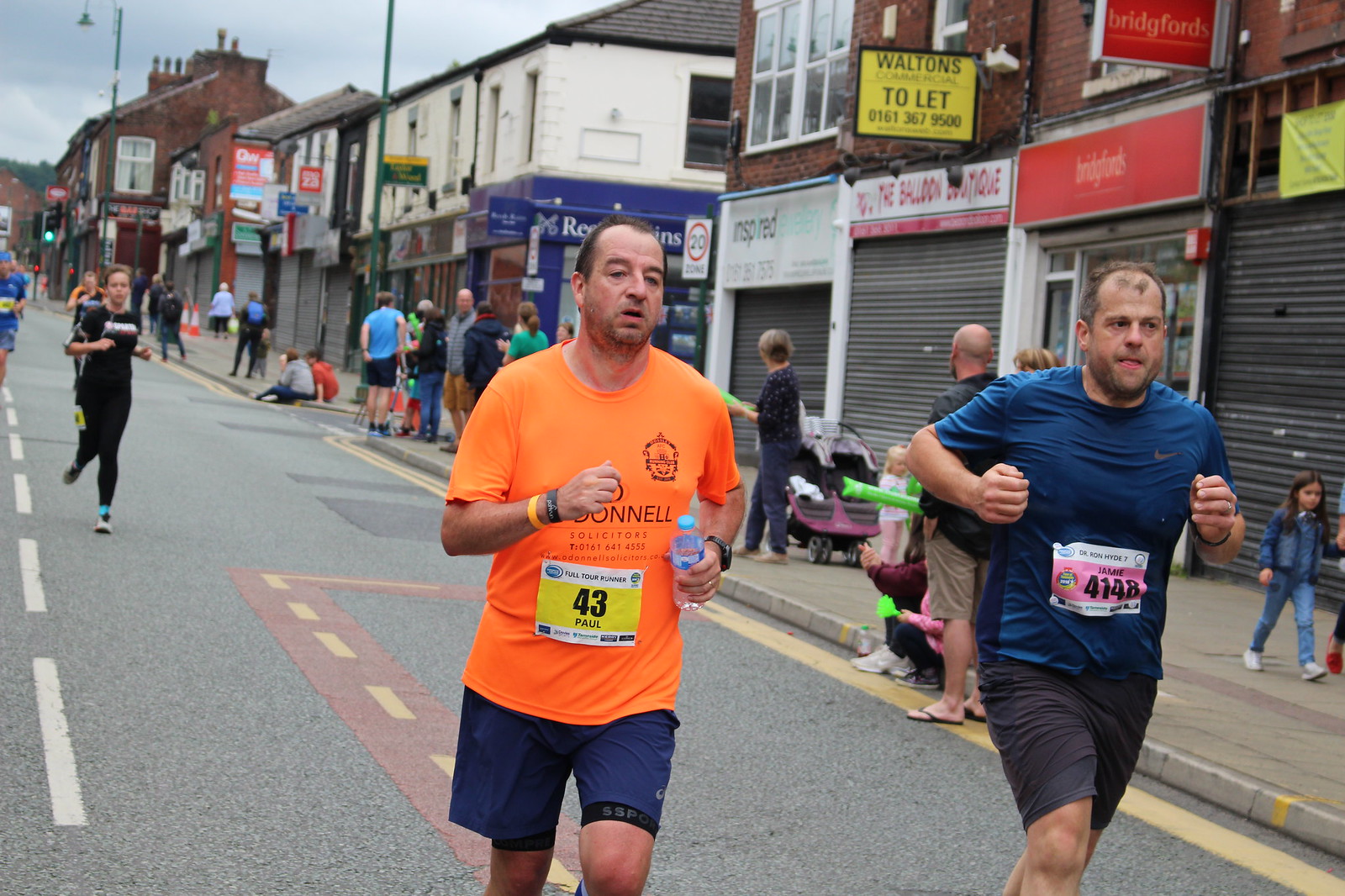The photograph captures an outdoor scene at what appears to be a street race happening in broad daylight. In the foreground, two men are running side-by-side down a road made of asphalt. The man on the left is wearing a bright neon orange t-shirt paired with navy blue shorts. Affixed to his chest is a runner's tag that reads "43 Paul" in black text on a yellow background. Beside him, a man in a navy blue Nike shirt and black shorts runs with a tag that reads "Jamie 4148" in black text on a pink and white background.

In the background, multiple runners can be seen racing down the street. The race is flanked by storefronts with corrugated metal doors pulled down, suggesting the stores are closed. Notable signs include one in red reading "Bridgeford's" and another in yellow with black writing that says "Walton's Toolette" followed by a phone number. Along the sidewalk to the right, spectators watch the race, some sitting while others walk by, often accompanied by children. The array of colors in the scene includes gray, white, maroon, orange, yellow, blue, and tan, contributing to the vibrant, bustling atmosphere of the race day.